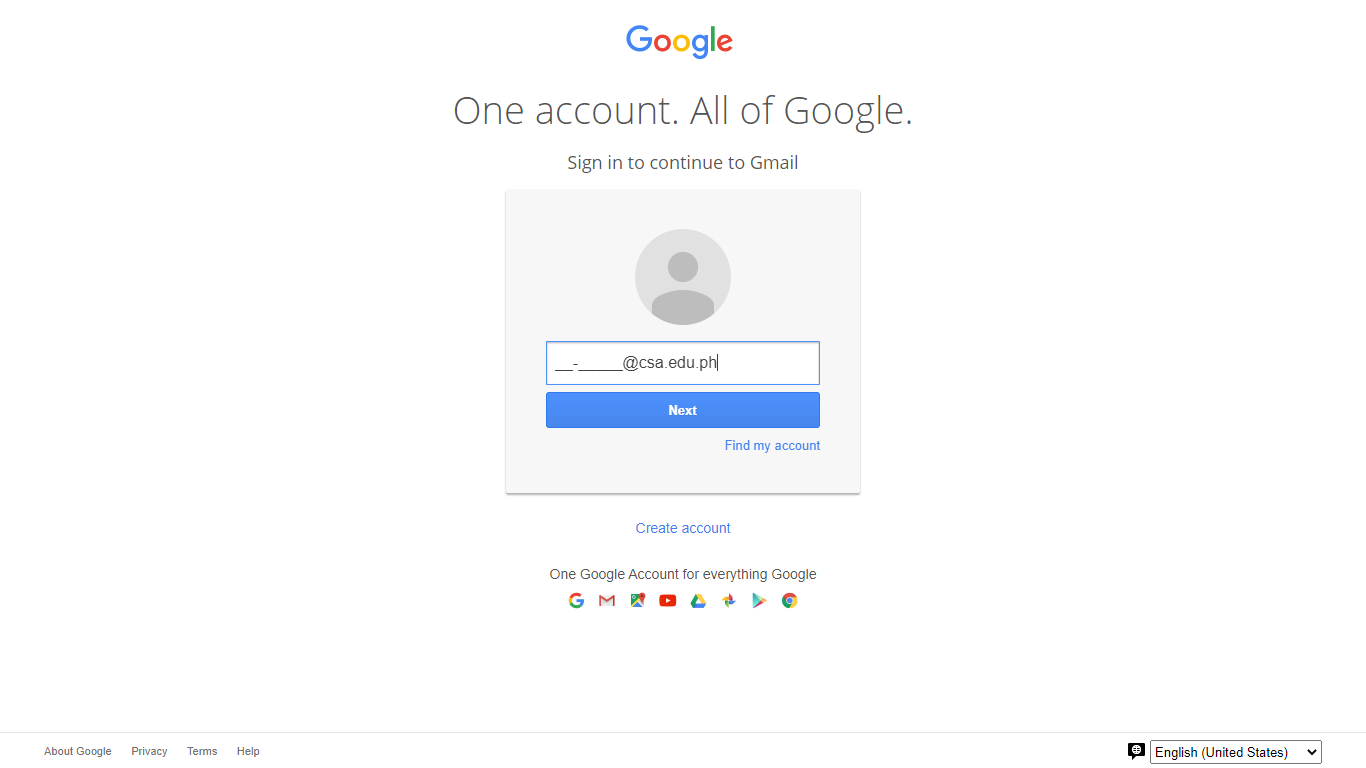The image appears to be a partial screenshot of a Google sign-in page on a mobile device. The top section of the screen is entirely white, prominently featuring the Google logo. The logo consists of a capital "G" in blue followed by lowercase letters: "o" in red, "o" in yellow, "g" in blue, "l" in green, and "e" in red. Beneath the logo, the text "One account. All of Google." is displayed in a very thin, tall, gray font.

Below this message, there's an instruction to "Sign in to continue to Gmail." Following this text, there's a gray rectangle containing a generic avatar icon—a simplified depiction of a head and body. Next to the avatar, there appears to be an incomplete email address input field: it shows a series of blanks, a hyphen, another blank, followed by "@csa.edu.ph", with the cursor still active, indicating that the email address is yet to be completed.

At the bottom of the gray rectangle, there's a blue button labeled "Next," intended to be clicked once the email input is complete. Below this button, options for "Find my account" and "Create account" are available. Finally, a footer message reiterates, "One Google account for everything Google," accompanied by various Google service icons, highlighting all the Google services accessible through a single account.